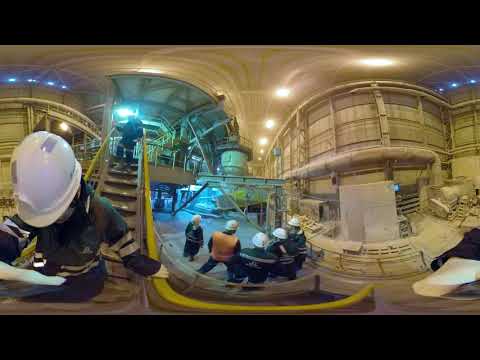The image captures a dynamic scene within a large, industrial warehouse or manufacturing plant, taken with a 360-degree panoramic view. The setting is bustling with activity, featuring workers clad in industrial protective gear. All visible personnel, identifiable by their white hard hats, are dressed in dark clothing accented with reflective high-visibility stripes. In particular, one individual dons an orange safety vest among the five workers congregated in the middle ground, engaged in a discussion and facing away from the camera.

Prominently in the foreground, a yellow-handled metal stairway descends, occupied by two individuals; one nearer to the top, dressed in black PPE, and another at the bottom, intently examining something in his hand, possibly a piece of paper. The expansive and structured environment is punctuated by complex industrial elements—pipes, steel girders, vents, and metal panels lining the walls—suggesting a well-equipped facility. Concrete and wooden slabs, along with other equipment, are visible towards the right. Overhead, the ceiling displays a network of lights and tubing controlling the illumination. In the distance, massive conveyor belts extend, poised perhaps for transporting metallic materials, underscoring the site’s industrial nature. The scene effectively showcases a robust, active industrial environment with a focus on worker safety and complex machinery.